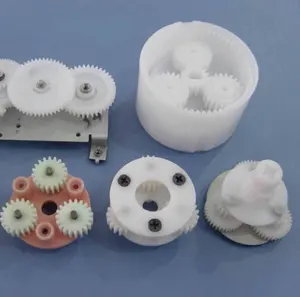The photograph showcases a collection of disassembled plastic cogwheels, laid out meticulously on a flat, light blue surface that appears to be a table or counter. The focal points include five distinct assemblies of gears, primarily white with grooved notches along the sides. 

In the top left corner sits a white and silver rectangular platform. This platform features a small bracket in its bottom right corner, hosting three larger white cogwheels affixed by bolts. directly to its right, there's a cylindrical white container holding three white cogwheels at triangular intervals within. Moving to the lower right, another assembly consists of a smaller white circular component stacked atop a larger gray one, each with its own set of cogwheels—white on top and gray on the bottom. 

Centered at the bottom is a circular object with three screws securing a flat white base, beneath which the wheels are positioned. In the lower left corner, a coral-colored base showcases three white cogwheels, each anchored by screws, and is distinguished by its three raised sections with small circles. Overall, the image presents these intricate mechanical components in a detailed and organized manner, emphasizing their structural diversity and plastic composition, reflecting the varied yet interconnected design of what might be parts of a machine or device awaiting reassembly.